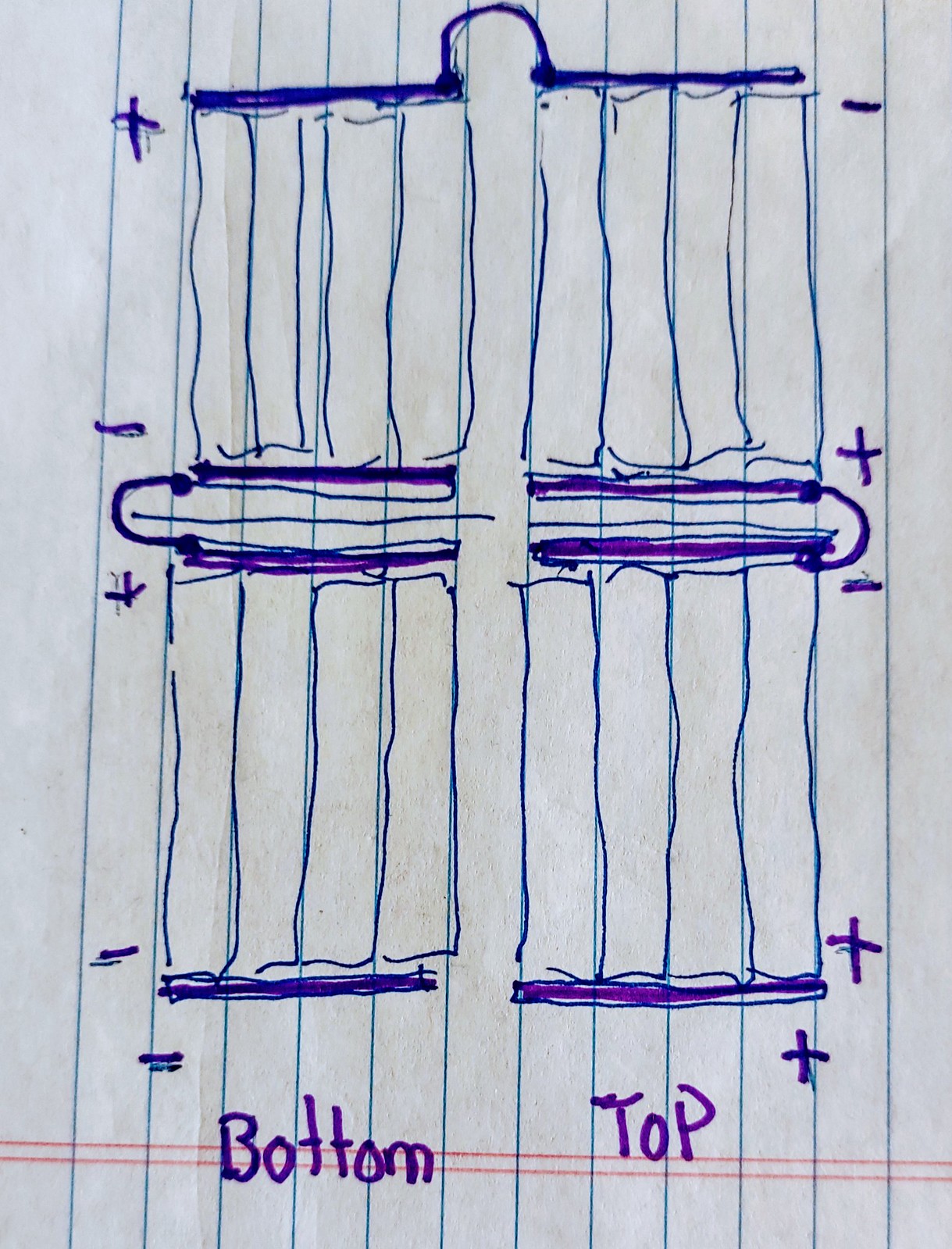A detailed sketch on vertically oriented lined notebook paper depicts a technical diagram, potentially representing an electrical circuit involving batteries. The teal-colored lines of the notebook provide a distinctive background, with two horizontally-oriented red lines running along what is now the bottom edge. The diagram, apparently drawn using pen and possibly marker, features a structured layout: four columns on the left separated by a space from four columns on the right, all connected at the top. A plus sign marks the left side, while a minus sign marks the right side, suggesting a polarity typically associated with batteries. At the bottom of the diagram, the columns appear again, this time inverted, with a plus sign at the top and a minus sign at the right. The bottom edge displays another minus sign on the left and a plus sign on the right, mirroring the upper portion of the sketch. The terms "bottom" and "top" are inscribed in purple marker, adding labeling to the intricate drawing.